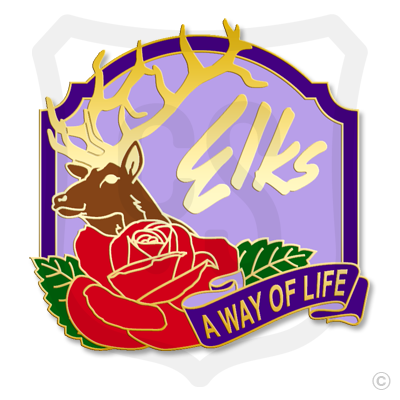The image depicts a detailed logo, centrally placed against a white background. The logo is reminiscent of a shield or squarish dome, encased in a gray outline that transitions into purple with a surrounding yellow border. Inside this emblematic design, a prominent, gold-outlined elk head, featuring gold horns and a brown face, stands out to the left. Adjacent to it on the right, the word "Elks" is emblazoned in matching gold. Beneath the elk's head, a red rose with green leaves and golden outlines is prominently displayed. Below this floral element, a purple banner featuring yellow text reads, "A Way of Life." The composition incorporates a variety of colors, including white, gray, brown, purple, light purple, red, green, and gold. Additionally, there's a copyright symbol located at the bottom right corner of the image. This logo, taking up most of the image, resembles what might be used for corporate branding on websites, business cards, or letterheads.